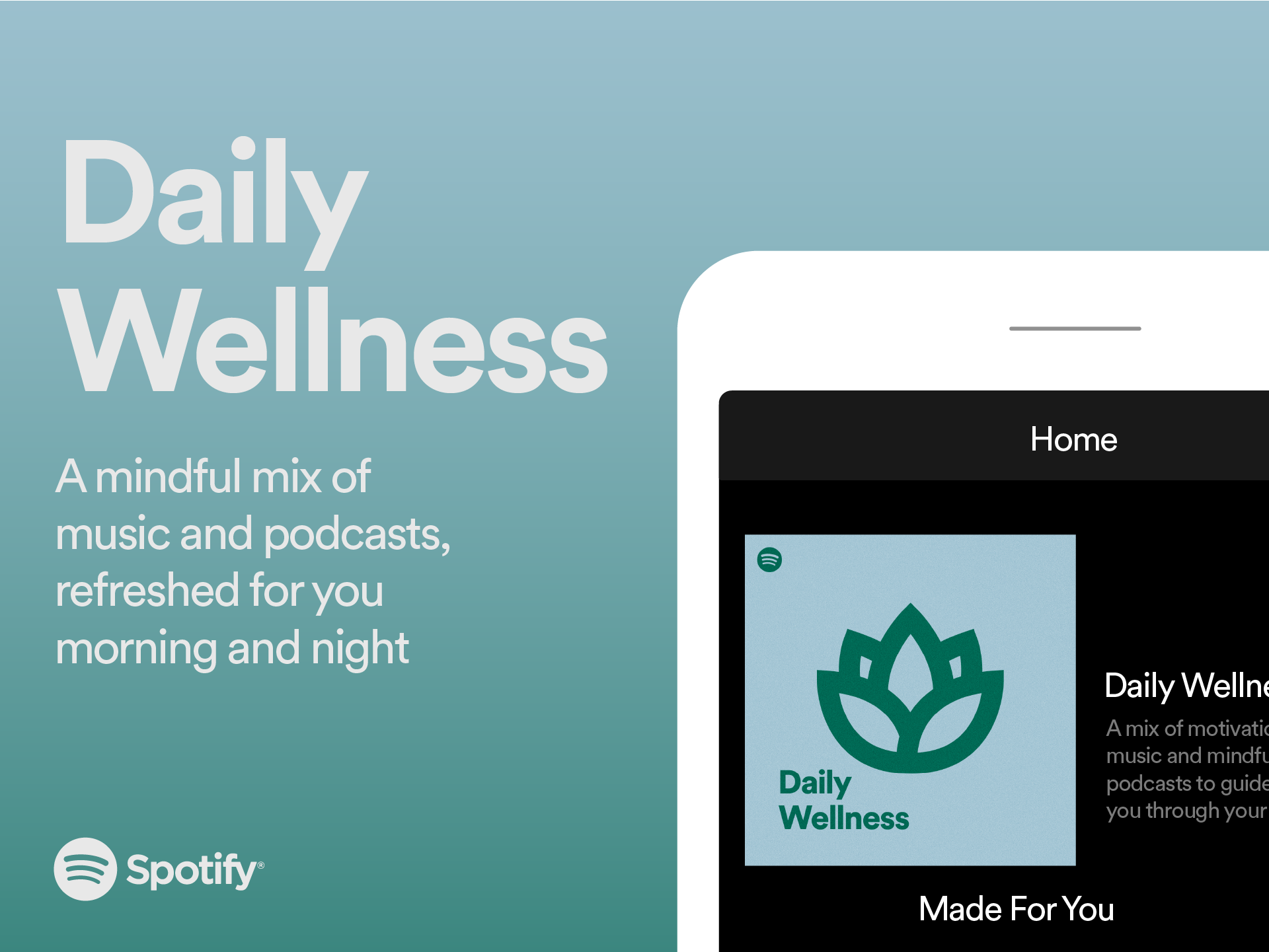Here is a refined and detailed descriptive caption based on the provided voice note:

---

"Featured on a soothing gray-blue background, this promotional image highlights Spotify's 'Daily Wellness' playlist. Positioned in the bottom right corner is a sleek white tablet displaying the 'Home' screen. The display shows a banner for 'Daily Wellness,' featuring a curated mix of motivational music and mindful podcasts designed to guide your day, refreshed every morning and night. The text on the banner reads 'Daily Wellness - A mix of motivational music and mindful podcasts to guide you through your day.' The background behind the banner has a gradient effect, transitioning from a darker shade at the bottom to a lighter hue as it ascends. In the bottom left corner, the familiar Spotify logo—a white circle with three curved lines—is prominently displayed against the background, symbolizing the streaming service's dedication to enhancing personal well-being through curated auditory experiences."

---